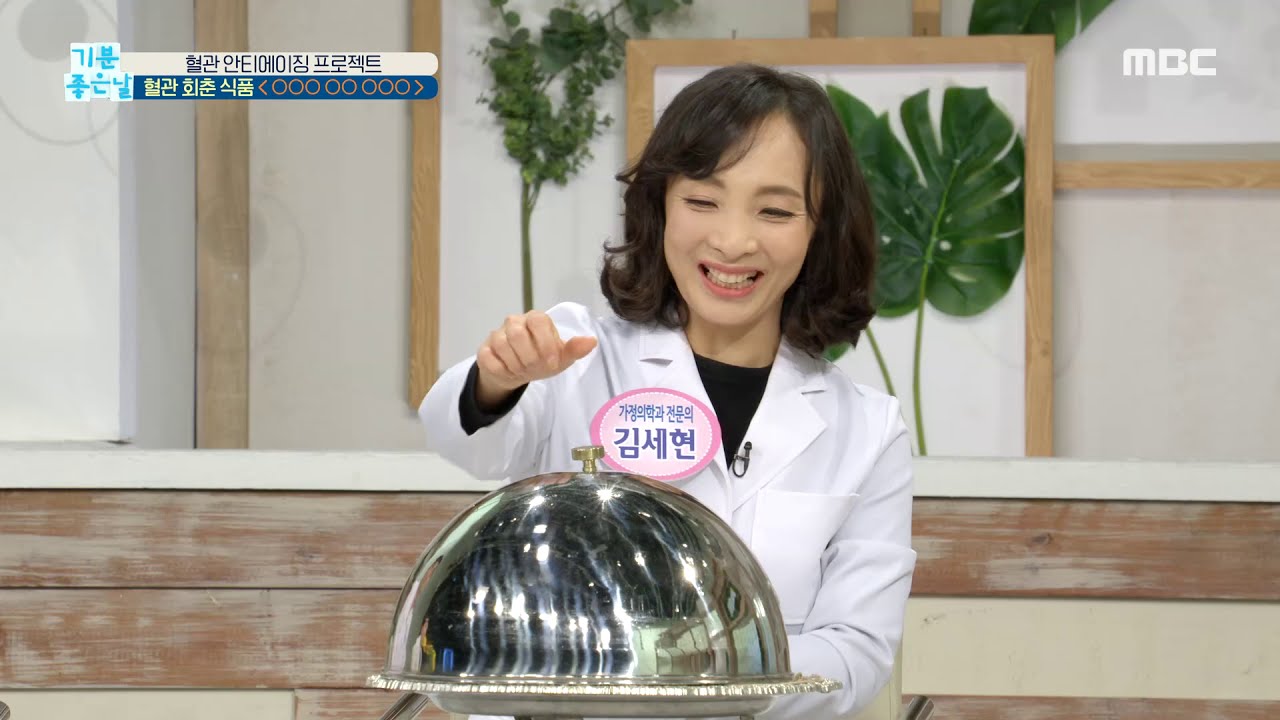The image depicts an Asian woman with a clear complexion and black hair, dressed in a white chef coat with a badge displaying Asian characters. She appears to be participating in a cooking contest or TV show, as she stands poised to lift a silver domed lid off a large dish in front of her. The setting features a wooden background with green leaves and floral elements, evoking a studio or staged environment. In the upper right corner, the white bubble letters "MDC" are visible, while the upper left corner features a navy blue and white banner with Asian writing and colorful accents. The scene suggests a blend of culinary expertise and television presentation against a distinctly styled backdrop.